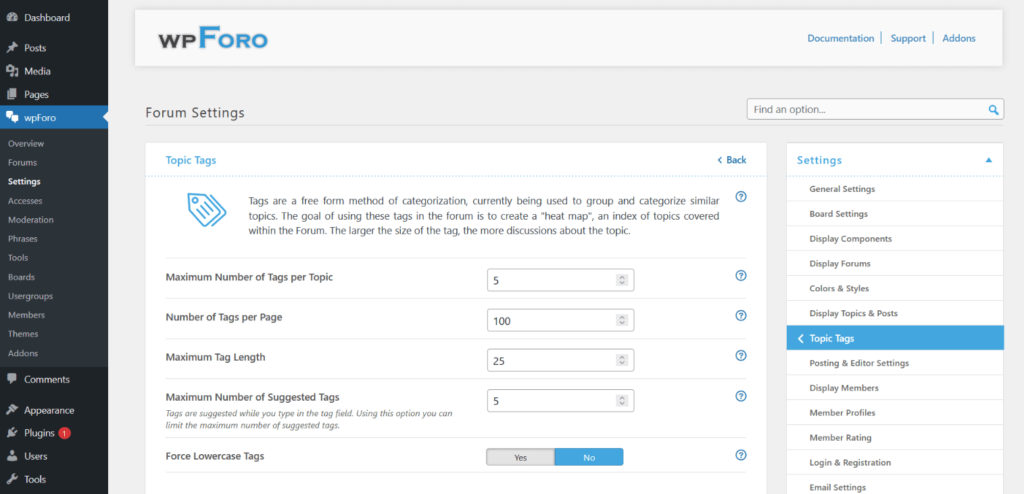The image features a user interface from a dashboard. 

On the left-hand side, there is a long rectangular menu. The top section of this menu has a bluish-gray background with the word "Dashboard" displayed in gray font. Below this, in smaller gray lettering, it lists several menu items: "Post," "Media," "Pages," and "WPForo." The "WPForo" item is highlighted, indicating it is the current selection, by a blue background and an arrow pointing left towards it.

Beneath "WPForo," the background color returns to gray with gray text listing "Overview," "Forums," and "Settings," the latter of which is slightly bolder and white. Following these, additional items include "Accessories," "Moderation," "Phrases," "Tools," "Boards," "User Groups," "Members," "Themes," and "Add-ons," presented in a similar style.

The lower section of the menu transitions to a black background, featuring "Comments" in white font, with smaller white texts for "Appearance" and "Plugins." A red circle with a white number one is positioned to the right of these items, indicating a notification. This section concludes with "Users" and "Tools" listed at the bottom.

In the middle of the page, the top section has a rectangular area with a white background. On the left, it displays "WP" in capital gray letters followed by "Foro," with the letter "F" capitalized and in light blue. To the right of this title, links for "Documentation," "Support," and "Add-ons" are written in blue, separated by vertical lines. Below this navigation bar, "Forum Settings" is written in gray, separated by a light gray divider.

The central area holds a square white background displaying blue text at the top left, reading "Topic Tags." Below this, there's a blue clip-art image of a tag. The tag contains three lines and a dot at its tip, and is oriented such that its tip points toward the upper left.

Overall, the layout and color usage offer clear navigation and accessibility within the dashboard interface.